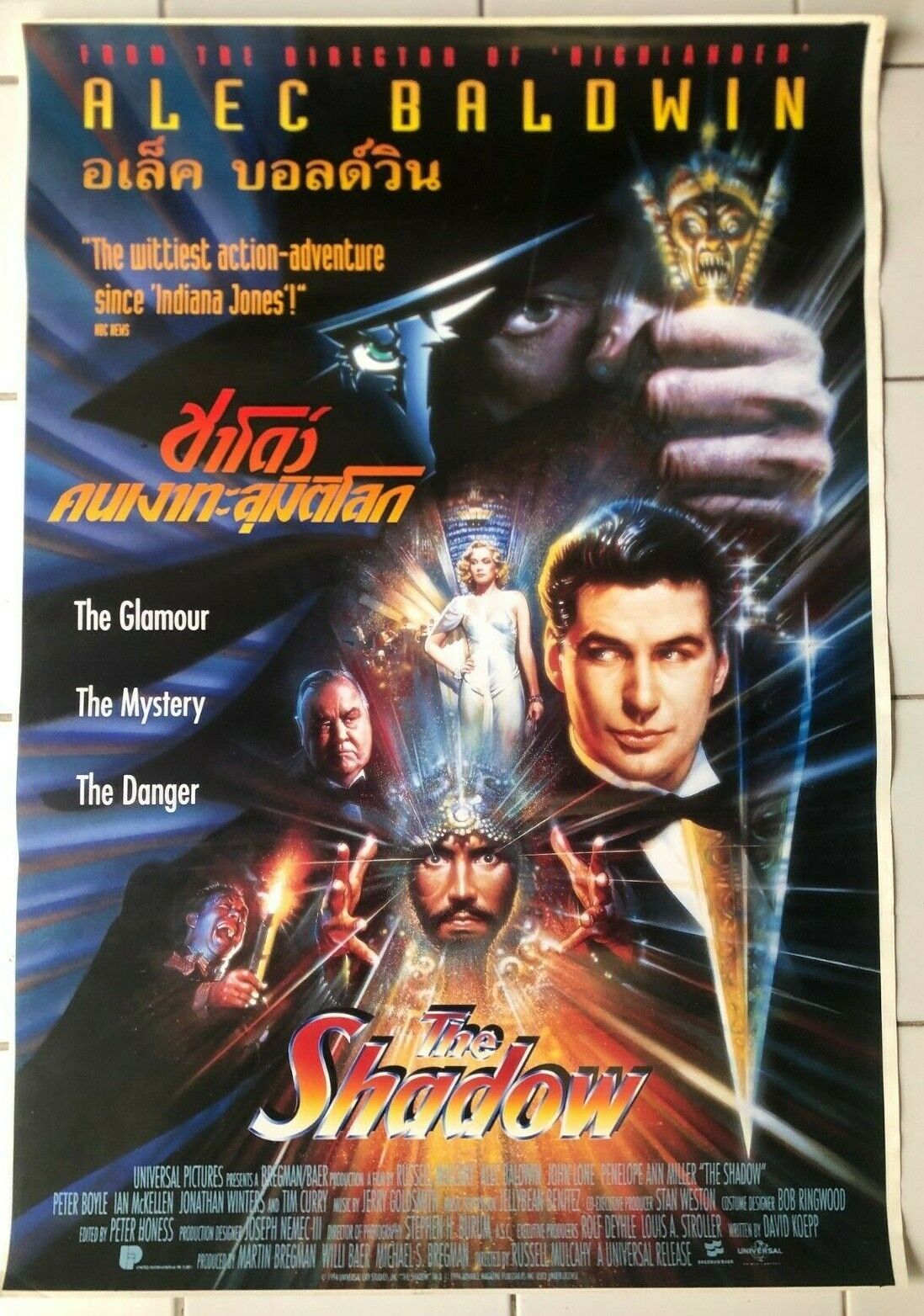This is an intricately designed movie poster for "The Shadow," featuring a prominently displayed Alec Baldwin. His youthful face dominates the top portion of the poster, framed by an ominous eye and a gold-colored medallion or wand held in a left hand, which has an archaic face on it. Below Baldwin's visage, there is a striking depiction of a woman dressed in white, exuding a sultry demeanor that captures the viewer’s attention. Positioned smaller than Baldwin, she is centrally located. Above the film’s title, "The Shadow," a mysterious male figure with piercing eyes framed by his hands and a crown-like headpiece is displayed; he appears to emit rays of light. Further adding to the intrigue is a gray-haired, older man on the left side, although his identity isn't clear. The background features a shadowy, cartoonish figure with veiled eyes and a black hat clutching a talisman in his left hand. Across the top, the name "Alec Baldwin" is emblazoned in yellow letters, followed by foreign script that suggests this poster might be intended for an international audience, possibly in Thai. The tagline "The wittiest action adventure since Indiana Jones" is displayed prominently, along with the phrases "the glamour, the mystery, the danger" in white lettering. At the bottom of the poster, "Universal Pictures" is listed alongside the standard credits for the film’s director, producers, and stars. The overall color scheme of the poster is quite dark, contributing to its moody and enigmatic atmosphere.